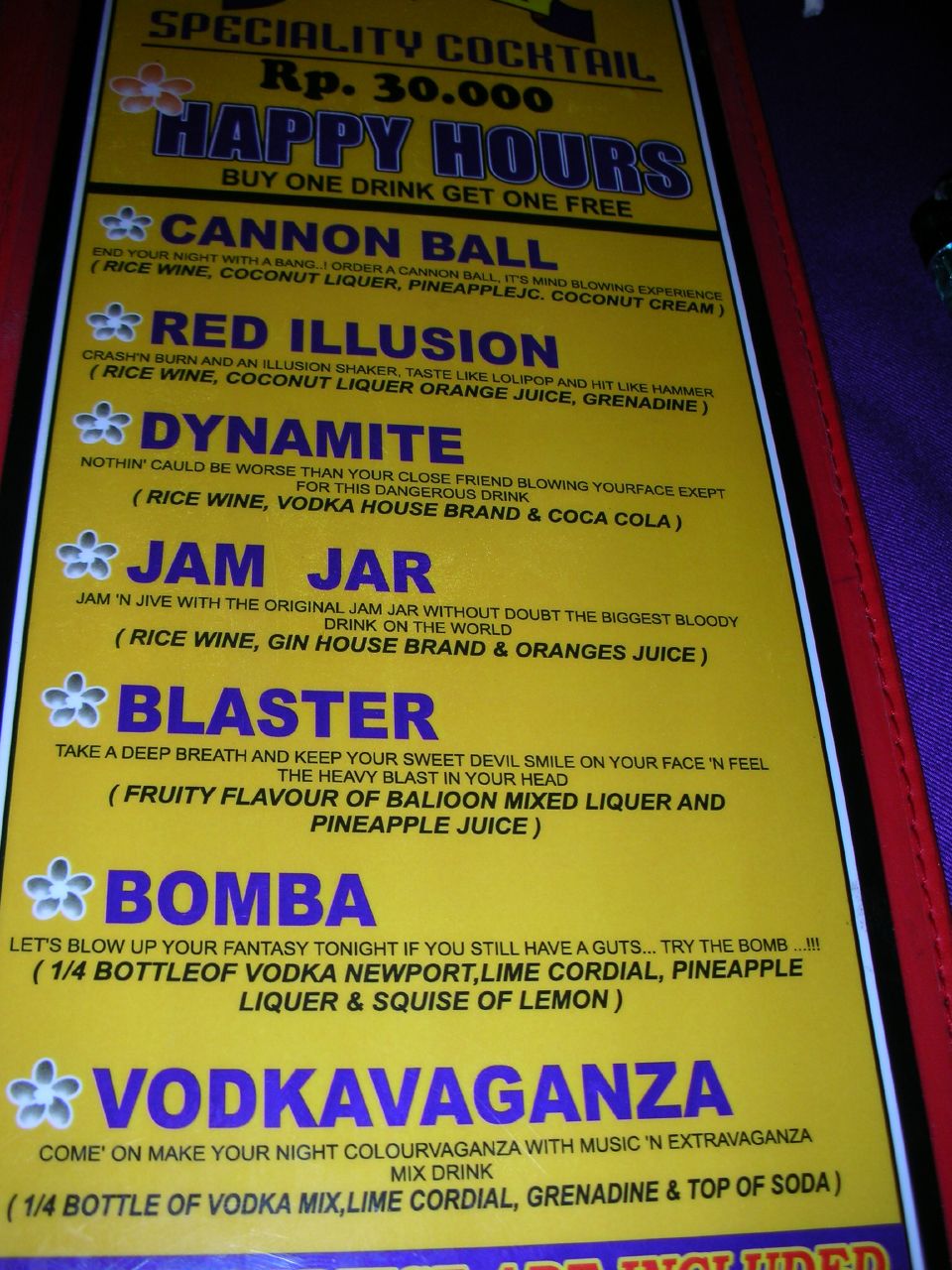This close-up photograph captures a tall yellow menu with a stitched red border and a blue background, possibly displayed outdoors in India, given the "RP 30.000" pricing. At the top, "Specialty Cocktail" is written in prominent black text, followed by "Happy Hour" in large blue letters underneath. Beneath the Happy Hour promotion, "Buy One Drink, Get One Free" is stated in black text. Below a black dividing line, the menu lists several specialty cocktails in blue capital letters, each accompanied by a small white flower to the left. The cocktails include Cannonball, Red Illusion, Dynamite, Jam Jar, Blaster, Bomba, and Vodka Vaganza. Detailed descriptions and ingredients for each drink are provided in black text under their respective names. The menu not only invites patrons to enjoy a variety of creative beverages but also promises a vibrant experience, blending music and an extravaganza of mixed drinks.